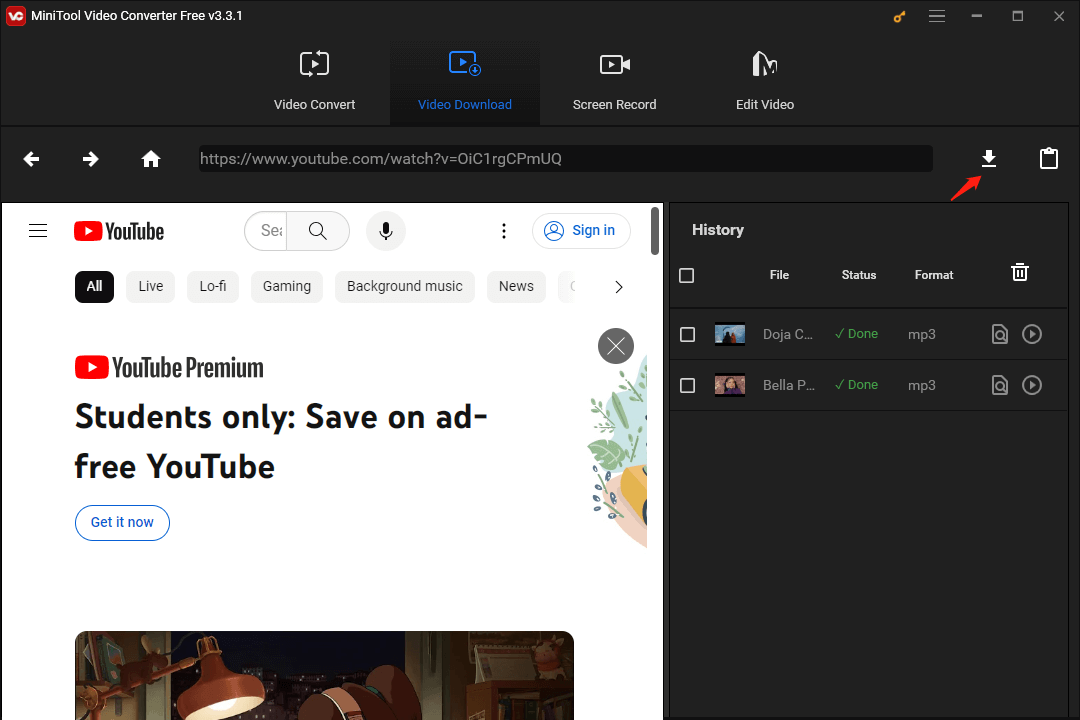The image displays the interface of the MiniTool Video Converter Free software. At the top left corner, the title "MiniTool Video Converter Free" is prominently displayed, accompanied by a red square icon with the letters "VC" inside it. To the right of this title, the main navigation options include "Video Convert," followed by an unreadable option due to it being highlighted in blue, "Screen Record," and "Edit Video," each with their corresponding symbols above.

Below this navigation bar, there are buttons that allow the user to navigate backward and forward, and a Home button written in gray. The webpage features a link to YouTube.com, serving as a direct access point for watching videos.

The central portion of the screen is dedicated to YouTube's interface. It showcases the YouTube logo, a hamburger menu, a search bar, and a microphone icon for voice search. There is also a "Sign Up" button. Directly below these elements, the navigation tabs are visible, with "All" being currently selected. Other options include "Live," "Lo-Fi," "Gaming," "Background Music," "News," among others. A promotional banner for "YouTube Premium" targeting students highlights savings and an "Ad-Free YouTube" experience with a "Get It Now" call-to-action.

On the right side of the screen, there is a history section set against a black background. Here, the user’s past interactions are listed, showing icons representing the content types, a brief description, the status, and the format, which are both labeled as mp3 files. Trash icons are available for users to delete items from the history.

This detailed interface offers a comprehensive overview of the capabilities and resources available within the MiniTool Video Converter Free software, intertwined with YouTube’s functionalities.